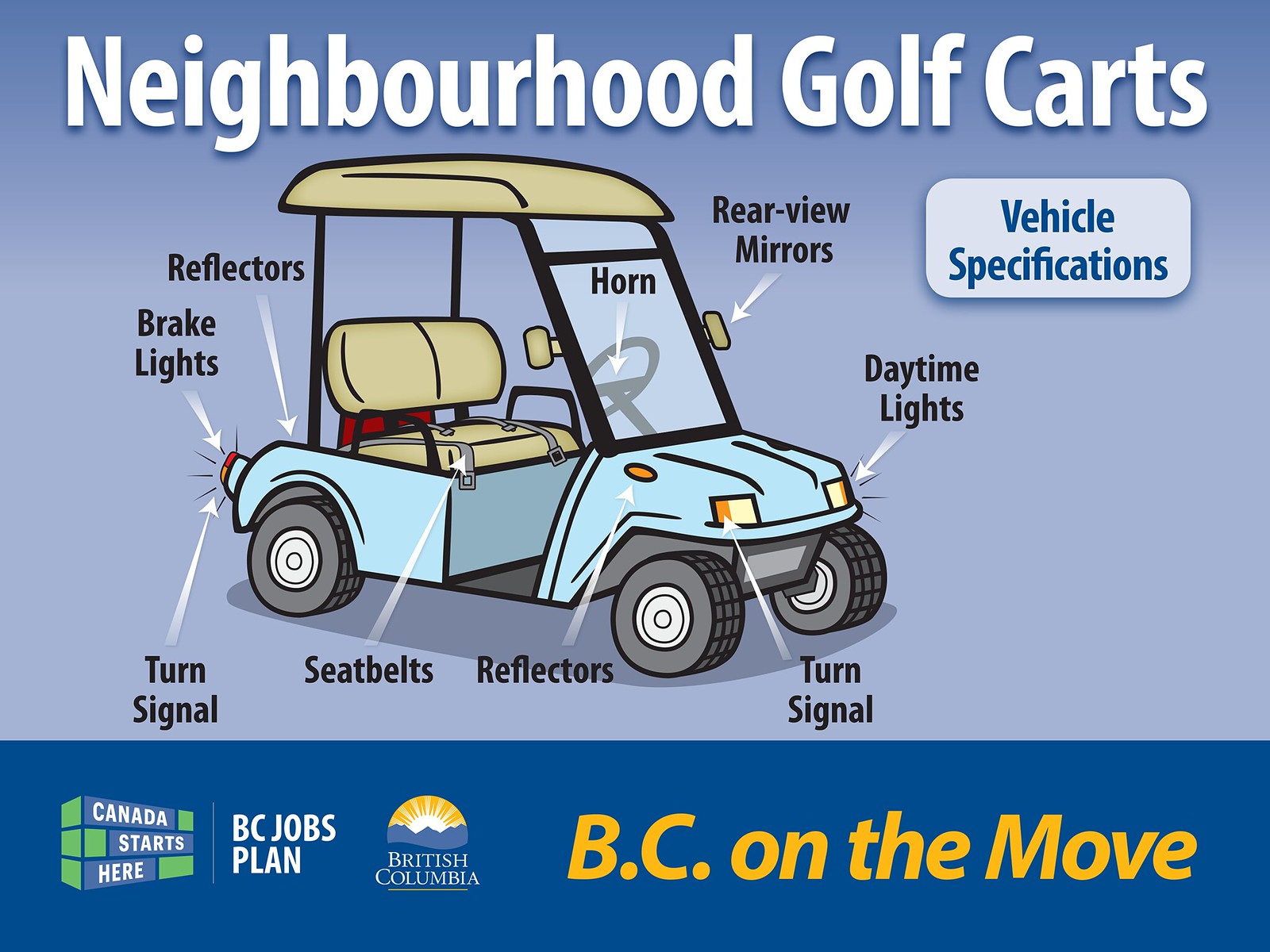This large, square infographic features a predominantly blue background, with a darker blue section at the bottom. Centered at the top in large, white sans-serif letters is the title "Neighborhood Golf Carts," accented with a soft dark blue shadow. Below the title is a detailed illustration of a light green golf cart with tan seats and roof. Various components of the golf cart are labeled with black text and indicated by white arrows, including reflectors, brake lights, turn signals (both front and back), seat belts, daytime lights, a horn on the windshield, and rearview mirrors.

To the upper right of the cart illustration, a white, rounded rectangular box labeled "Vehicle Specifications" provides a blueprint of the vehicle. The text within this box matches the dark blue color and font style used throughout the infographic.

At the bottom, against the dark blue section, several logos and text elements are displayed. On the left, the logos for "Canada Starts Here," "BC Jobs Plan," and "British Columbia" are grouped together, the latter featuring a design with a mountain range and radiating yellow sunbeams. To the right, in large, bold yellow letters, the text "BC On The Move" is prominently featured.